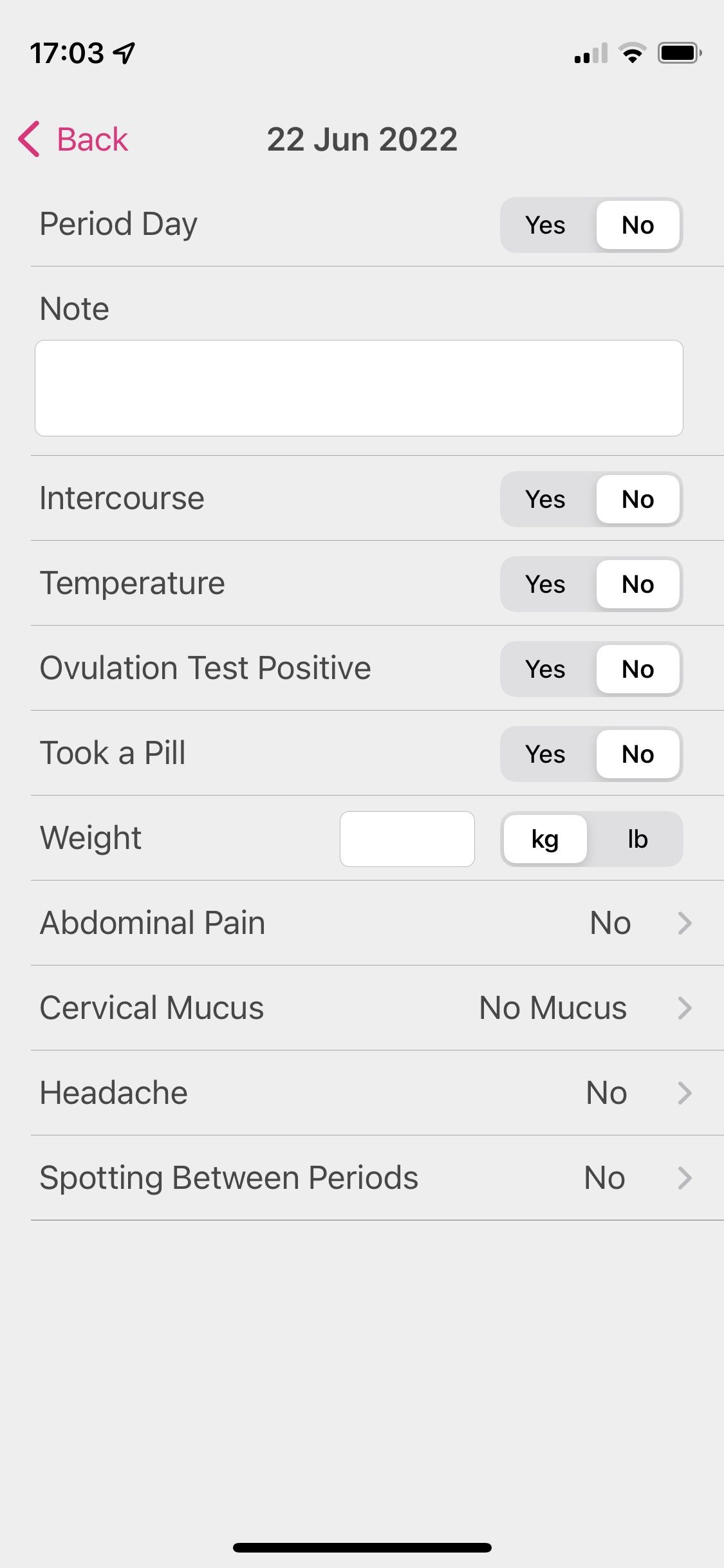This image is a screenshot taken in portrait mode from a cell phone. The background is predominantly gray, and the screenshot appears to display a form interface. In the upper left-hand corner, the timestamp reads "17:03," while the upper right-hand corner indicates a full battery. Below this, there is a pink back arrow labeled "Back" on the left side and, in bold text, the date "22 June 2022."

The form includes several toggle buttons for various options, each with choices of "Yes" or "No." The specific sections and their respective inputs in the form are as follows:

- **Period Day**: "No" is selected.
- **Note**: This section is currently blank.
- **Intercourse**: "No" is selected.
- **Temperature**: "No" is selected.
- **Ovulation Test Positive**: "No" is selected.
- **Took a Pill**: "No" is selected.
- **Weight**: This field is to be filled in with options for kilograms or pounds.
- **Abdominal Pain**: "No" is selected.
- **Cervical Mucus**: "No Mucus" is selected.
- **Headache**: "No" is selected.
- **Spotting Between Periods**: Unspecified in this description.

Though initially described as a pregnancy tracker, it is actually an ovulation tracker designed for a woman who is trying to conceive. The form appears thorough and user-friendly.